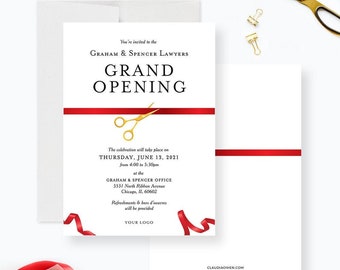This digital poster prominently features an invitation card-style design for the grand opening of "Graham and Spencer Lawyers." The central focus is a vertical, rectangular card with text in black, announcing the "Grand Opening." Below this, contact information is provided, though the details are difficult to read due to the small, compressed text. A vibrant red ribbon, being cut by a golden pair of scissors, adds a ceremonious touch to the design, symbolizing the grand opening event. Additional red ribbons adorn the bottom left and right corners of the card, enhancing the celebratory theme. Behind this card, a white-colored back view with another ribbon and a grey envelope are visible. The background of the poster is light grey with some scattered, indistinct text in various colors. A visible date mentions Thursday, June 11th, enhancing the event details. This intricate combination of elements results in a refined, yet busy, visual emphasis on the grand opening celebration.